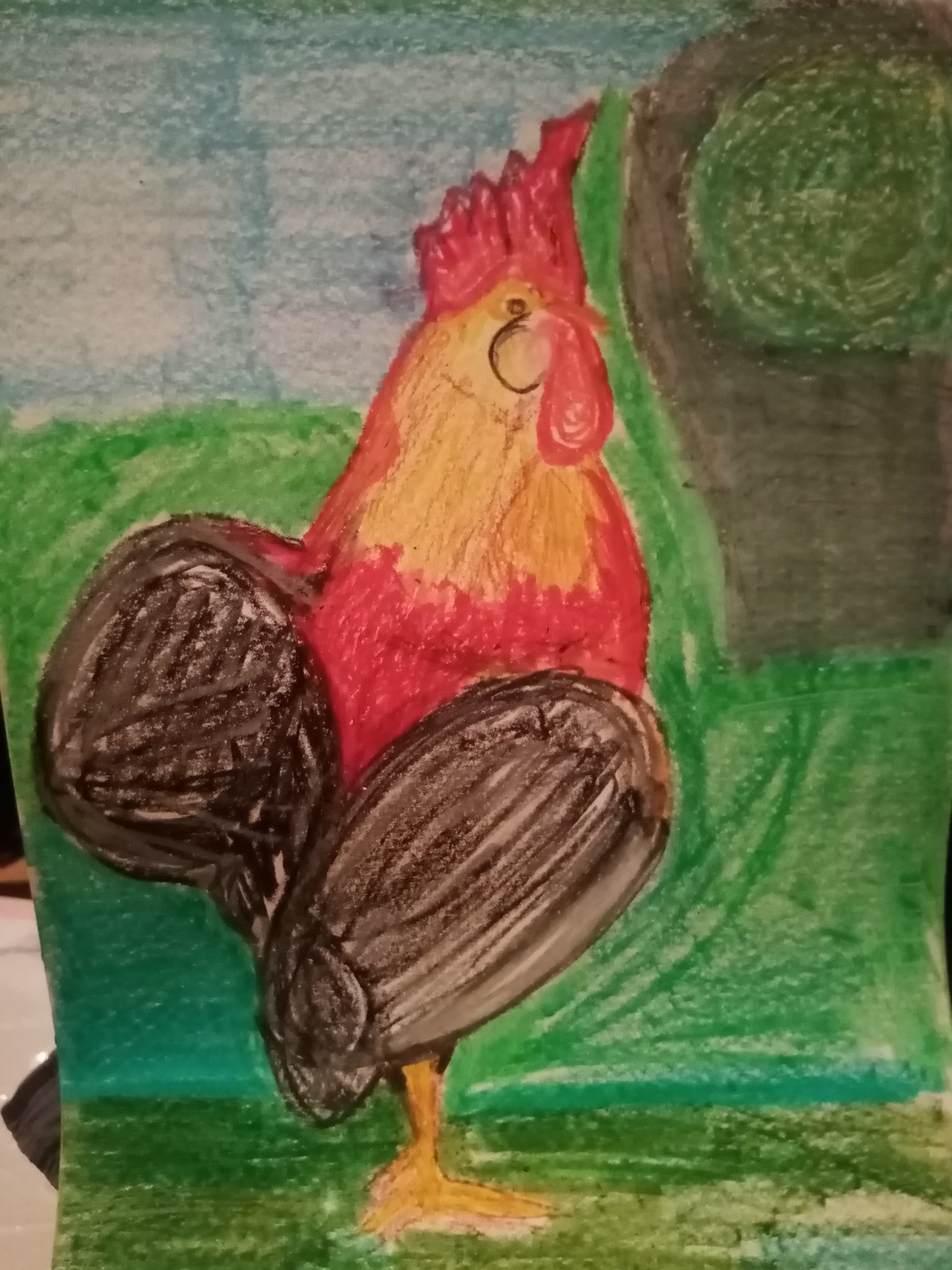This is a photograph of a detailed crayon or colored pencil drawing that features a vibrant, somewhat unrealistic rooster. The rooster, viewed from the side, has a striking red color with a patch of orange over its head and down its neck, and a red crest resembling a mohawk. It also has a red wattle hanging from its chin and a black eye. The rooster's body is a mix of yellow and red, while its wings are black and white. It stands on green grass, with a background consisting of a blend of blue sky and various green hues, possibly depicting bushes or hedges. There is an ambiguous black and green object next to the rooster, which might represent a tree drawn with childlike simplicity. The rooster also has yellow feet. The overall scene is colorful and embodies a playful, whimsical artistic style.